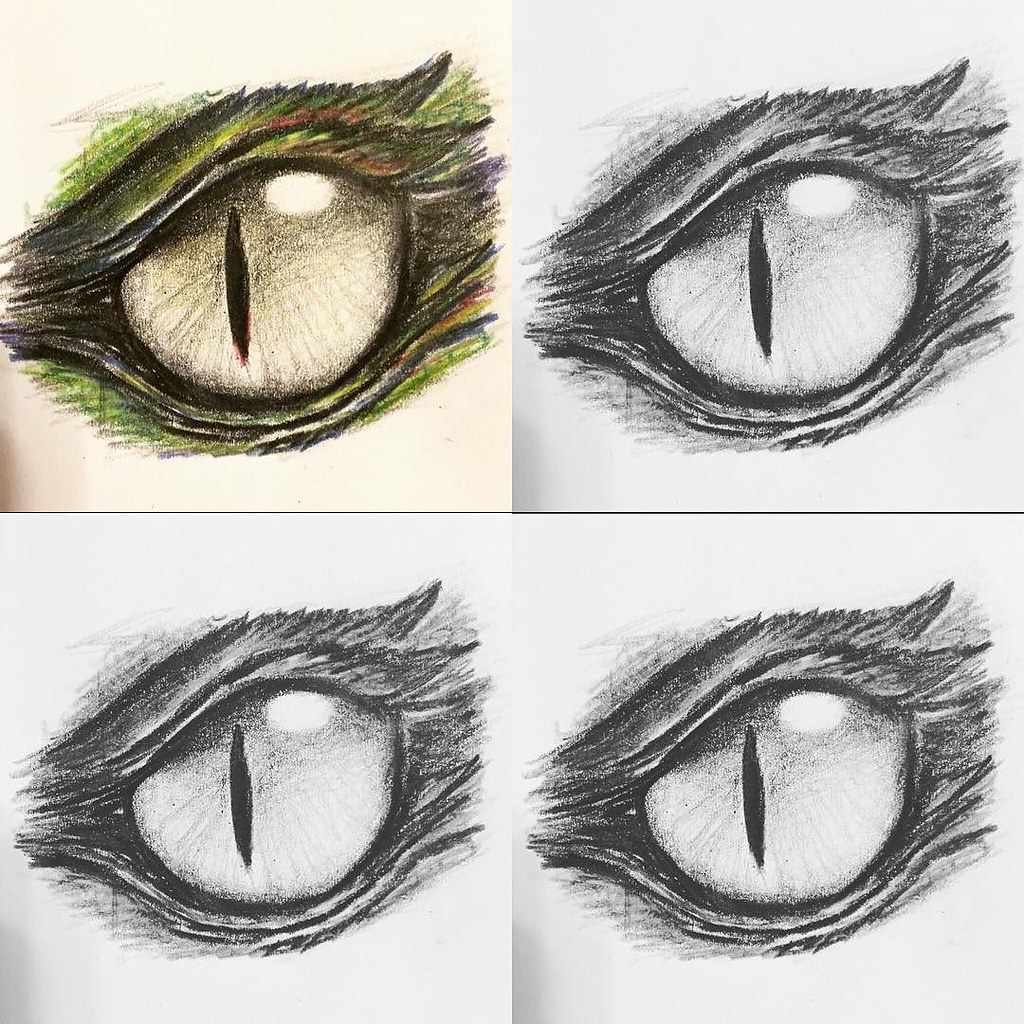The image is divided into a grid of four blocks, each displaying a detailed sketch of a dragon’s or reptilian eye at different stages of completion. The top left block features the most detailed and colorful version, drawn on a beige background. This eye has a green iris with yellow and white highlights, and a black slit pupil. The eye is framed by scaled eyelashes in shades of black, green, purple, and blue, adding a frowning appearance as the upper part is partially covered by an eyelid-like scale.

The top right block is a black-and-white version of the first eye, retaining all the intricate details without the color. The bottom left block shows a smaller version of the top right sketch, with the eye opened slightly wider and a simpler line work. Finally, the bottom right block presents the least detailed and most open version of the eye, with fewer feathers and scales, but maintaining the characteristic slit pupil and greenish tint around the edges. The progression highlights the transformation from an initial outline to a fully realized and vividly colored eye.